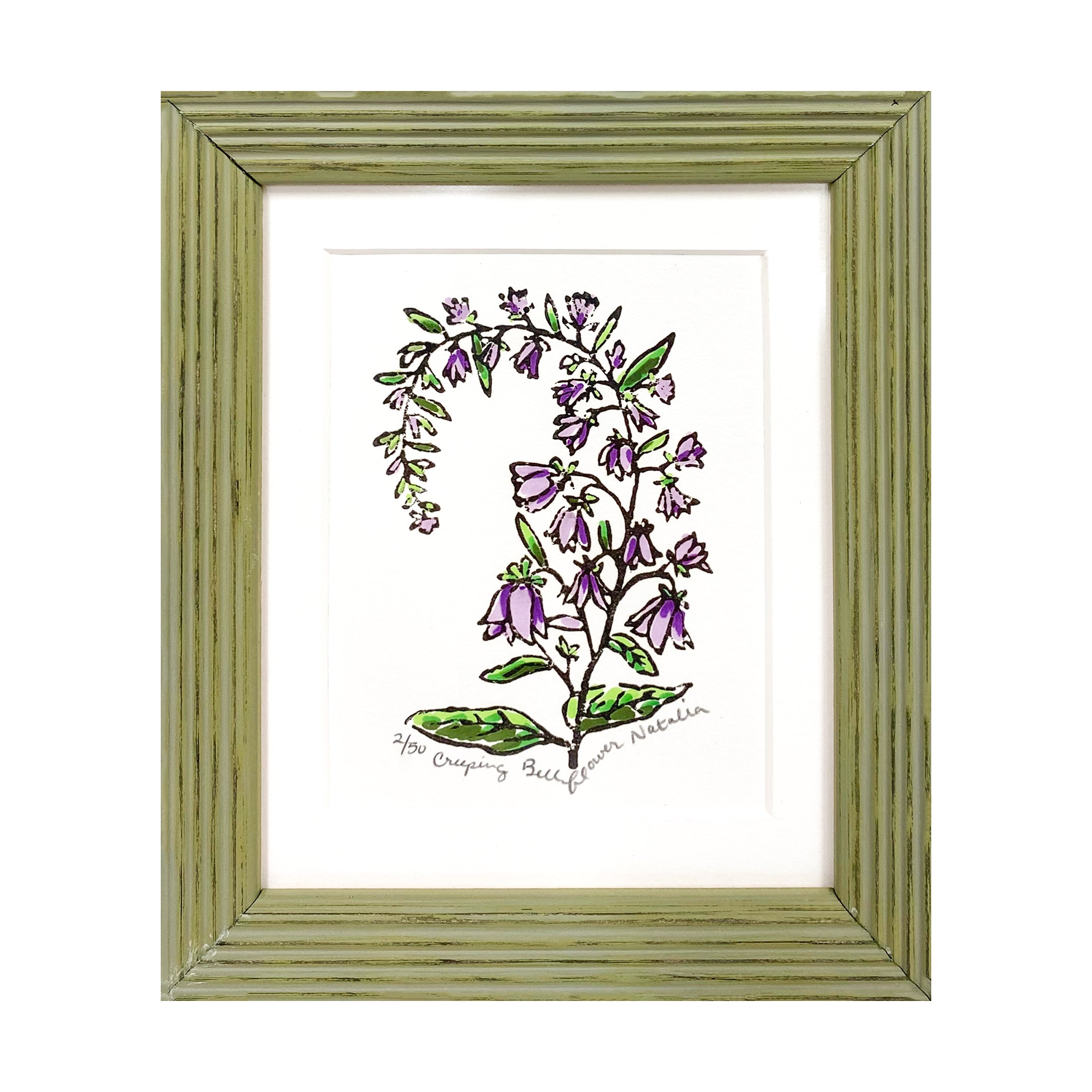The image showcases a simple yet vibrant drawing of a plant with lavender-colored, bell-like flowers and green leaves, presented on a white background. It features a light green, ridge-textured frame complemented by a double white or cream-colored mat. The plant itself, identified as a creeping bellflower, has a long, curved stem resembling a backward question mark, with flowers that appear in varying stages of bloom—some fully open and others still budding. The detailed illustration, potentially hand-drawn, gives off a delicate and elegant appearance, making it suitable for home display.